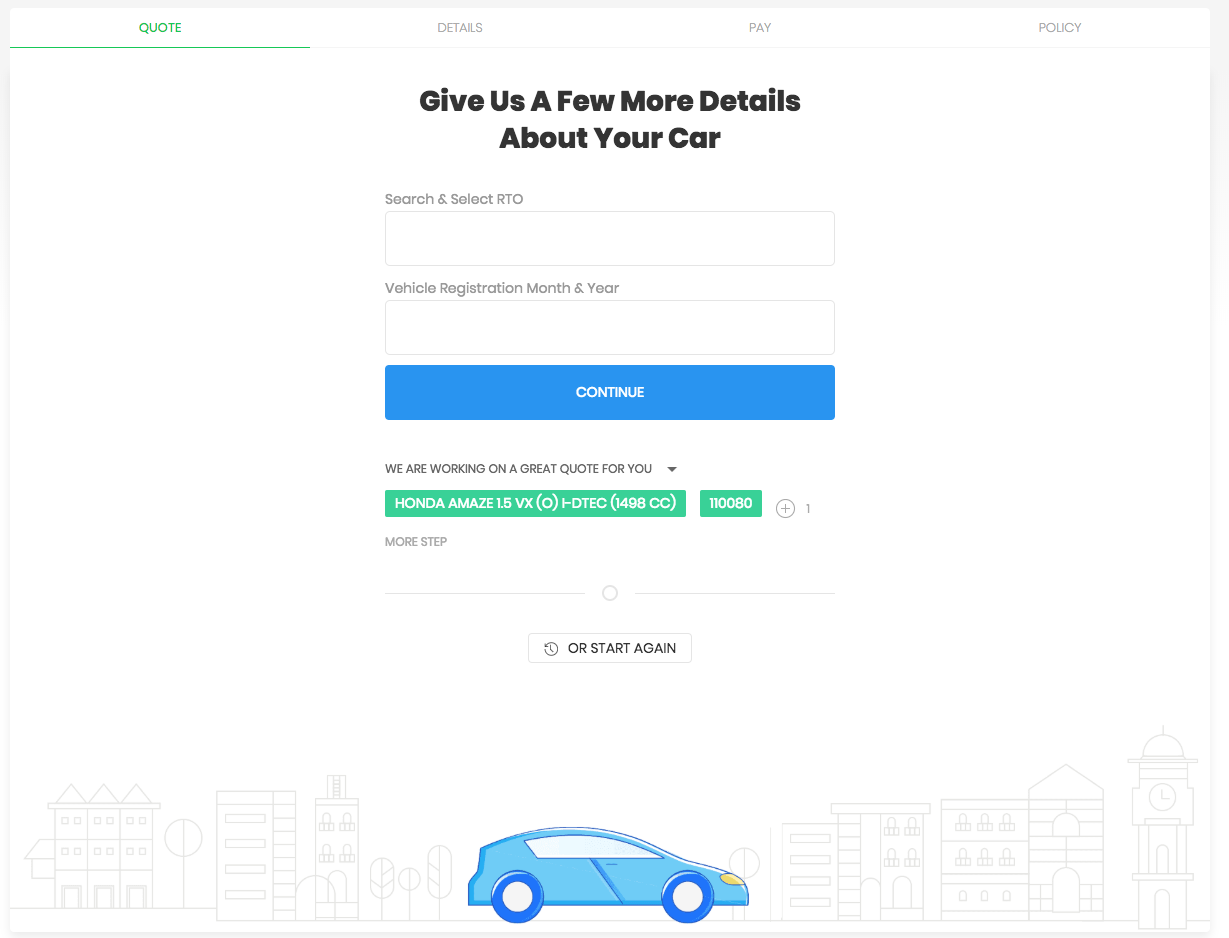Screenshot of an online car selling platform

The screenshot showcases an online platform designed for obtaining quotes for selling a car. The interface predominantly features a clean, white background. At the top of the screen, there are four columns with drop-down menus labeled: "Quote," "Details," "Pay," and "Policy."

Beneath these columns, a prominent message in bold, dark black letters reads, "Give us a few more details about your car." Directly below this message, two interactive pop-up boxes are visible. The first box prompts users to "Search and select RTO," and the second box asks for the "Vehicle registration month and year."

Below these fields, there is a large blue rectangle with white text that instructs users to "Continue." After entering the required information and clicking this button, the platform apparently retrieves specific details about the car. This is evidenced by a green highlighted box that appears, displaying the retrieved information about a particular car, although this detail occurs off-screen in the described process.